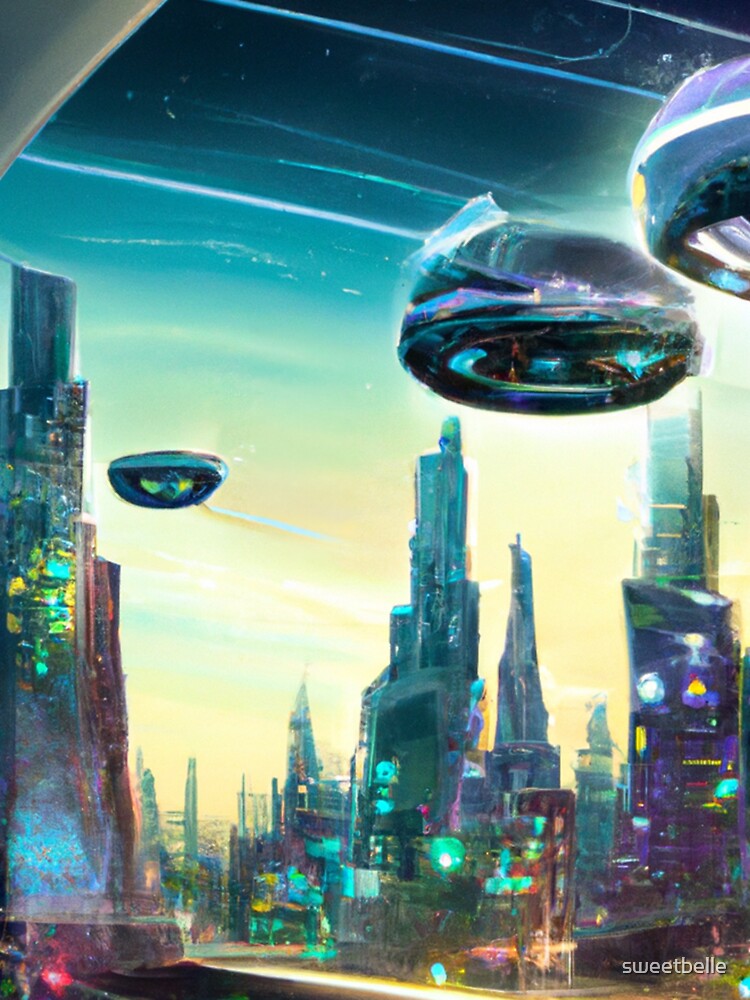The image depicts a vibrant, futuristic cityscape reminiscent of something out of a science fiction movie, comic, or game. Dominating the scene are tall, oddly shaped buildings in an array of colors including greens, blues, yellows, pinks, and purples. The city is aglow with scattered lights, enhancing the surreal atmosphere.

In the foreground, three circular flying objects, possibly small flying saucers, float through the air. These blue and turquoise crafts have pink and blue highlights, with black windows. One of them appears to be ascending into the sky, while the others maneuver near a building. 

The sky is a swirling blend of blue, green, yellow, and occasional pink hues, creating an otherworldly backdrop for the scene. In the lower right corner, the word "Sweetbell" appears as a single word, adding an enigmatic label to this ultra-modern urban fantasy. A large fountain on the left side of the image adds to the overall whimsical and imaginative setting.